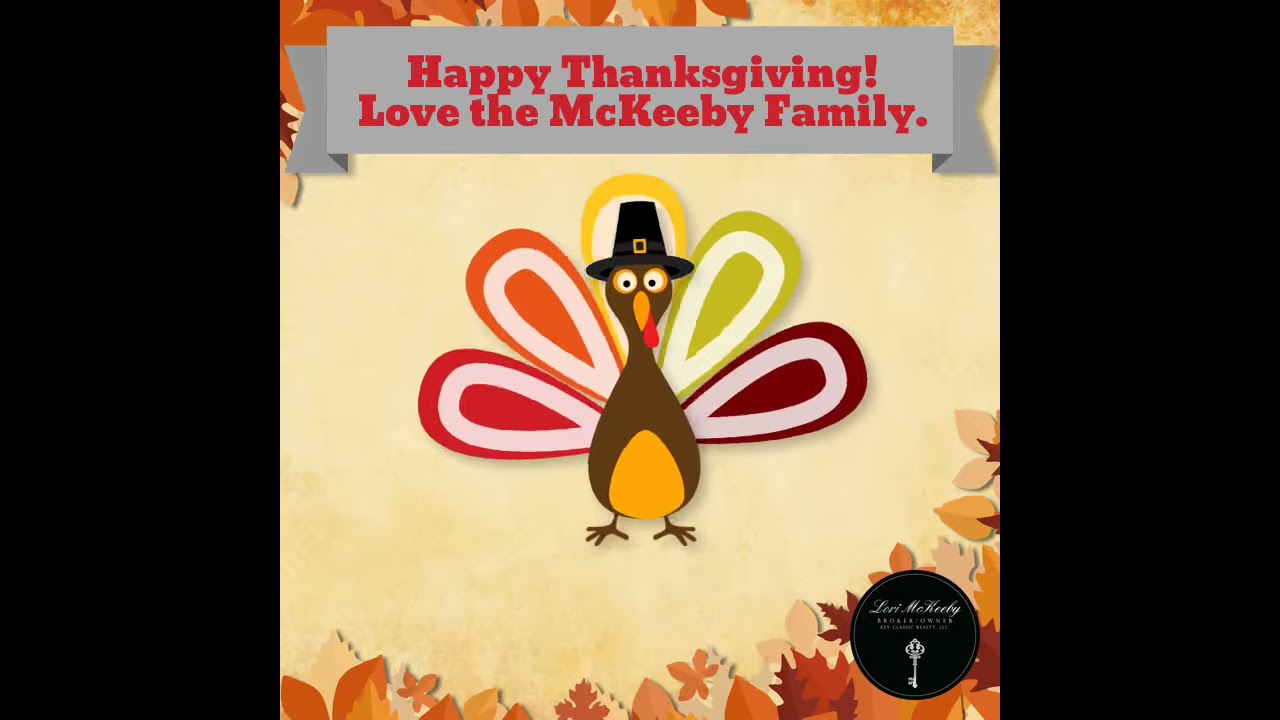This image features a cheerful, cartoonish turkey craft set against a beige background, flanked by two black vertical bars on either side, in a horizontally rectangular frame. The turkey, sitting prominently in the center, is adorned with five colorful tail feathers in red, orange, yellow, green, and maroon, each with a white oval design. It sports a black pilgrim hat with a buckle, has a brown body with a yellow belly, brown feet, a red waddle hanging below its beak, and expressive white eyes with black pupils encircled by a yellow line. Encircling the artwork are various autumnal leaves in shades of orange and brown. At the top of the image, a gray banner with red text reads, "Happy Thanksgiving. Love, the McKeebee family." In the lower right corner, there is a black circle featuring the text "Lori McKeebee, broker, owner," accompanied by an image of a key.